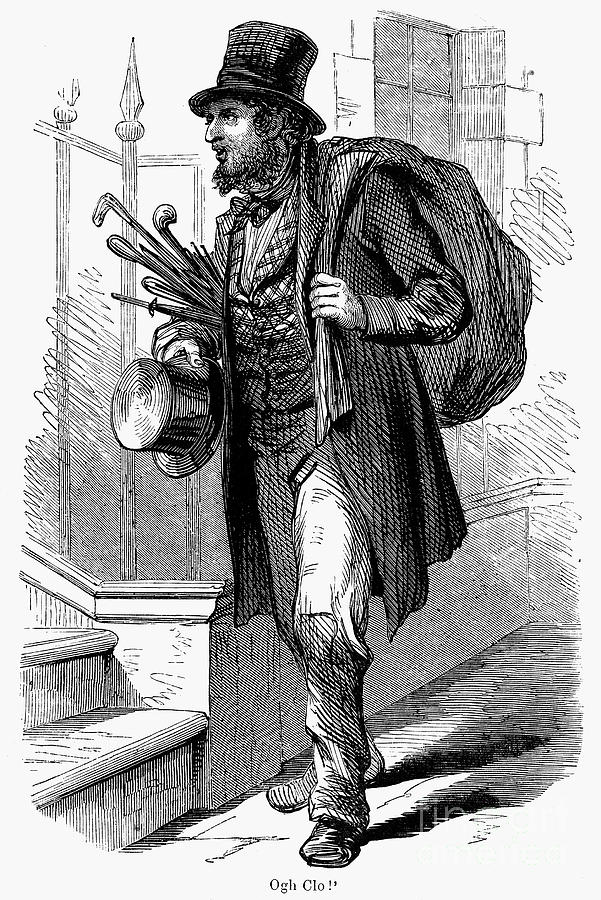The black and white pen-illustration depicts a man dressed in early 19th-century attire, evocative of a traveling salesman or possibly a street beggar. He is outfitted in a long coat reaching his knees, pants, shoes, and a jacket, with a scarf-like tie wrapped around his neck. He wears a top hat and carries a large sack over his left shoulder. In his right hand and under his arm, he holds another top hat filled with various sticks, canes, or pokers, one resembling a golf club. The man stands in front of a stone wall, adjacent to a set of steps and a metal fence topped with pointed bars. A building is faintly visible in the background, adding context to the scene.